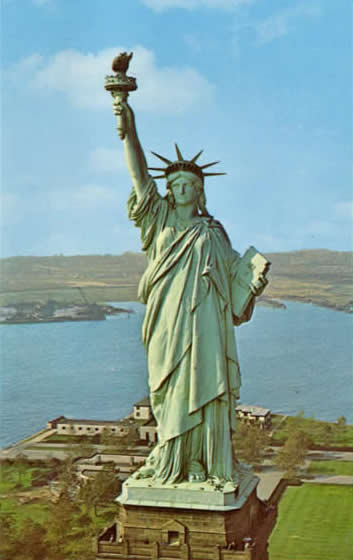This vertically rectangular, full-color aerial photograph captures a mostly sunny day with natural light, featuring the iconic Statue of Liberty. The image, likely taken from a helicopter, provides an eye-level view of the statue's face. The Statue of Liberty, with its characteristic greenish tint, stands prominently on a pedestal surrounded by a fence that includes visible doors. She holds a torch high in one hand and a book in the other, while adorned with her signature spiky crown. 

Below, the well-maintained grass and some trees cover the grounds of Liberty Island. Additional buildings dot the scene, with a large body of bluish water—the Hudson River—extending vertically through the center towards a distant landmass. This adjacent land, with its blend of brown and light-colored dirt, suggests an agricultural landscape, perhaps New Jersey. The horizon features a blue sky dotted with a few fluffy white clouds, adding to the composition's serene yet grand atmosphere.